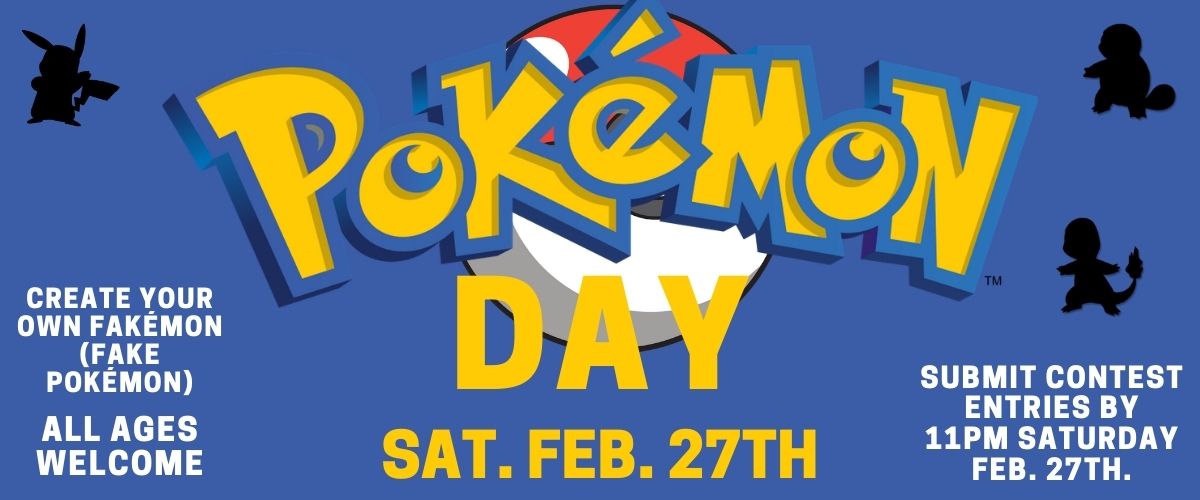This vibrant and meticulously designed banner promotes "Pokemon Day" with an eye-catching layout that features the signature playful Pokemon font. A large Pokeball serves as an engaging backdrop, highlighting the silhouettes of three beloved Pokemon: Squirtle, Charmander, and Pikachu. The banner announces that Pokemon Day will be celebrated on Saturday, February 27th, and emphasizes the deadline for contest entries, which must be submitted by 11 PM on the same day. The theme for this year is to create your own "Fakemon"—a fan-designed Pokemon, inviting participants of all ages to showcase their creativity. The overall design of the banner is visually appealing, ensuring it captures the attention of spectators and effectively communicates the event's details and excitement.